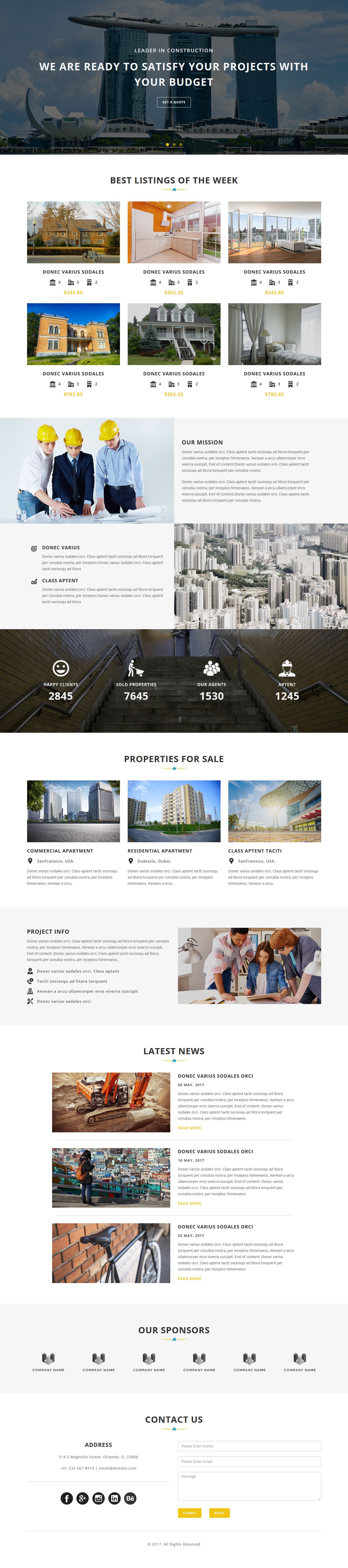The image is vertically oriented, roughly three times higher than it is wide, showcasing a compressed view of a website. The top 10% of the image features a semi-transparent banner overlaying an outdoor photograph. This photograph depicts multiple commercial buildings set against a partly cloudy sky. White text on the banner declares, "We are ready to satisfy your projects with your budget," with smaller, illegible text beneath it.

The main body of the image has a white background, displaying a centered line of black text which is too small to read. Below this text are six distinct images, each accompanied by three buttons. The images predominantly display various residential properties, including interior rooms and exterior views of homes. This section suggests a focus on real estate or home renovation.

At the mid-point of the image, on the left side, there are photographs of three men wearing yellow construction hats, implying a construction site context. Beneath these images are four additional pictures set against a gray background. The specifics of these images and any accompanying text are not discernible due to the reduced size.